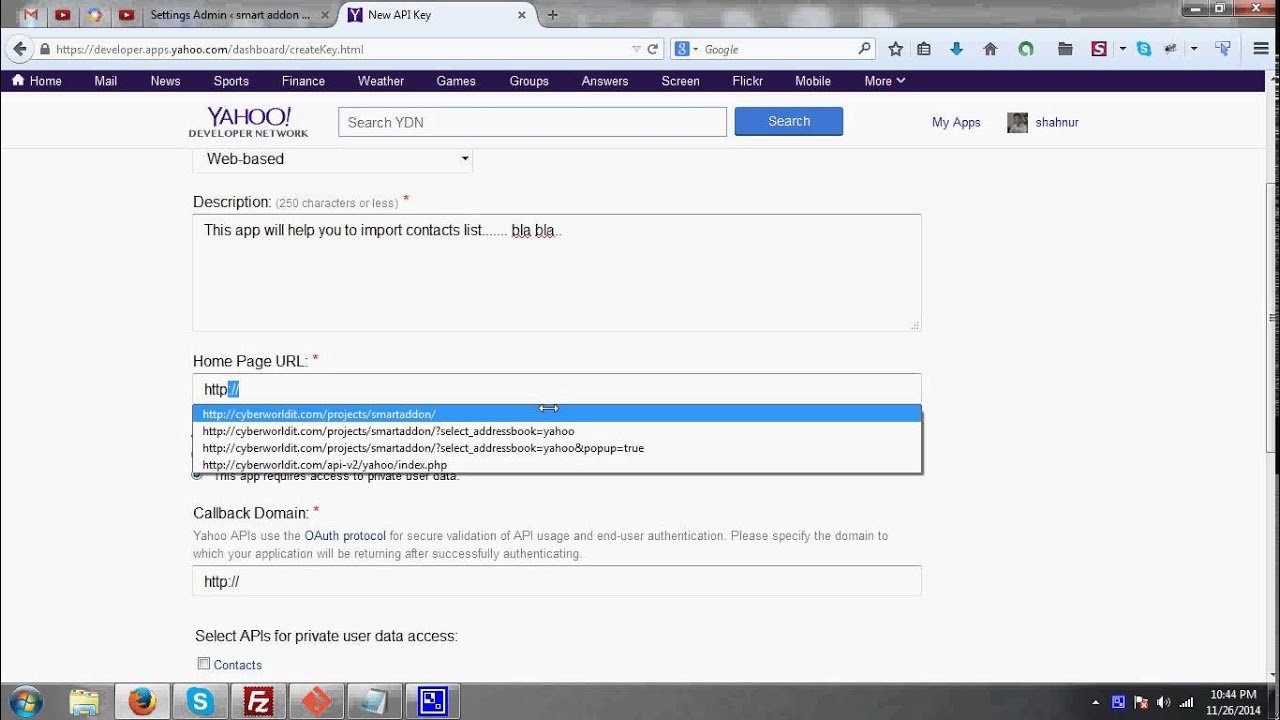The image showcases the home screen for the Yahoo Developer Network (YDN) displayed on a Windows computer. At the top of the window are the typical Windows taskbars, immediately followed by Yahoo's signature dark purple taskbar stretching across the entire screen. This bar, with its white font, features various options including Home, Sports, Finance, News, Weather, and Games, alongside a "More" button which unlocks additional menu items via a drop-down list.

Below this primary navigation bar, the screen prominently indicates that the current section is the Yahoo Developer Network. Adjacent to this label is a dedicated search box labeled "Search YDN," followed by a blue search button inscribed with the word "Search" in white. Beneath this, there is another input field designed to aid in more descriptive searching. The interface is rich with information and various tools, catering specifically to the needs of developers.